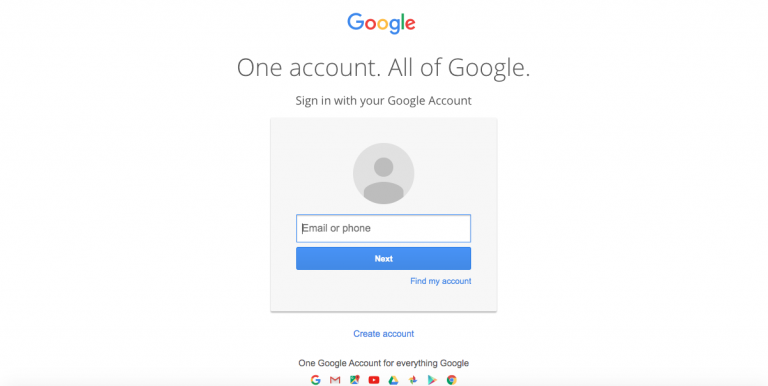The image depicts a screenshot of a mobile Google login page against a white background. At the top, the iconic Google logo, adorned in its vibrant rainbow colors, is prominently displayed. Directly beneath the logo, a dark gray text reads, "One Account, all of Google." Following this is an instruction to "Sign in with your Google account."

Located centrally on the screen is a light gray square. Within this square at the top, there is a placeholder for a profile picture, represented by a generic gray silhouette of a person. Below this placeholder, a text box is provided for the user to input their email or phone number, followed by a blue "Next" button with white text. Directly underneath this button, a link reads, "Find my account."

Beneath the prominent gray square is an additional white field. At the top of this section is a blue link labeled "Create account." Just below, a statement in dark gray text says, "One Google Account for everything Google." This is followed by an array of icons representing various Google services and apps, including Gmail, YouTube, Google Drive, the Play Store, and Chrome.